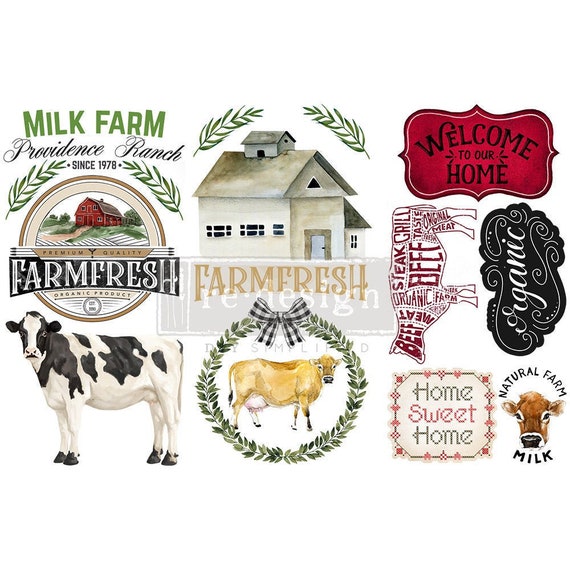The image is a detailed collage of advertisements and illustrations connected by the overarching theme of a farm named "Farm Fresh." Predominantly, the image is themed around "Milk Farm Providence Ranch" established in 1978. The main logo is prominently displayed, featuring the text "FARM FRESH" in all caps and situated above an idyllic red, two-story farmhouse with leafy ornamentation, set amidst expansive pastures.

Surrounding the farmhouse illustration, there are various farm-themed visuals: three cows depicted from different angles in black and white, light brown, and dark brown hues. Additionally, there's a cross-section diagram of a cow labeled with terms like "beef," "steak," and "grill," emphasizing the organic nature of the products. 

In the upper left corner in green text, the words "Milk Farm" appear, followed by the cursive text "Providence Ranch since 1978," accompanied by a leaf symbol. Below this, a black and white cow illustration is detailed, leading towards a separate drawing of a farmhouse with "FARM FRESH" text beneath it, encircled by a decorative green wreath with another cow illustration.

There are several text signs dispersed throughout the image, including "Welcome to Our Home," "Home Sweet Home," and "Natural Farm Milk," each adding to the homey, rustic ambiance. Additionally, there's a black and white sign declaring "Organic" along with a red, black, and white sign repeating the welcome message. Each detail combines to present a holistic and nostalgic advertisement for the Farm Fresh brand, celebrating organic farming and high-quality produce since 1978.